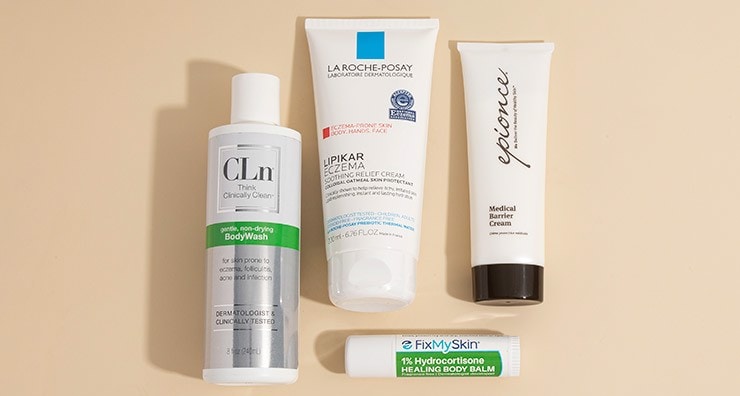The photograph captures a neatly arranged display of four skincare products on a light beige background, each item casting a shadow to its left. The products are laid flat in a rectangular landscape format, about two and a half times as wide as it is high. From left to right:

1. **CLN Thick Clinically Clean Body Wash**: Presented in a cylindrical tube with a smaller cap, this product features a distinctive design with the brand name "CLN" in large capital letters on a light gray upper section. Below a green band reading "Gentle Non-Drying Body Wash" is a silver lower section filled with smaller text.

2. **La Roche-Posay Lipikar Eczema Soothing Relief Cream**: This is a white squeeze tube slightly flatter in its profile, with "La Roche-Posay" prominently displayed at the top. The middle of the tube reads "Lipikar Eczema Soothing Relief Cream," emphasizing its purpose as an eczema treatment.

3. **Medical Barrier Cream**: Appearing to the right, this product is housed in a smaller cylindrical container with a black cap and an off-white body. Near the bottom, it bears the label "Medical Barrier Cream" and features a brand name that appears to start with a "P" or "EP," written in cursive at an upward angle.

4. **Fix My Skin 1% Hydrocortisone Healing Body Balm**: Positioned horizontally at the bottom of the arrangement, this white container has "Fix My Skin" in blue at the top and a green bar in the middle containing the description "1% Hydrocortisone Healing Body Balm."

Together, these products—each with distinct packaging and labeling—represent a variety of skincare solutions aimed at maintaining skin health, from body washes and creams to specialized balms. The clear and attractive arrangement of the items allows easy reading and recognition, replicating the style of product displays commonly found on e-commerce platforms like Amazon or Google Shopping.